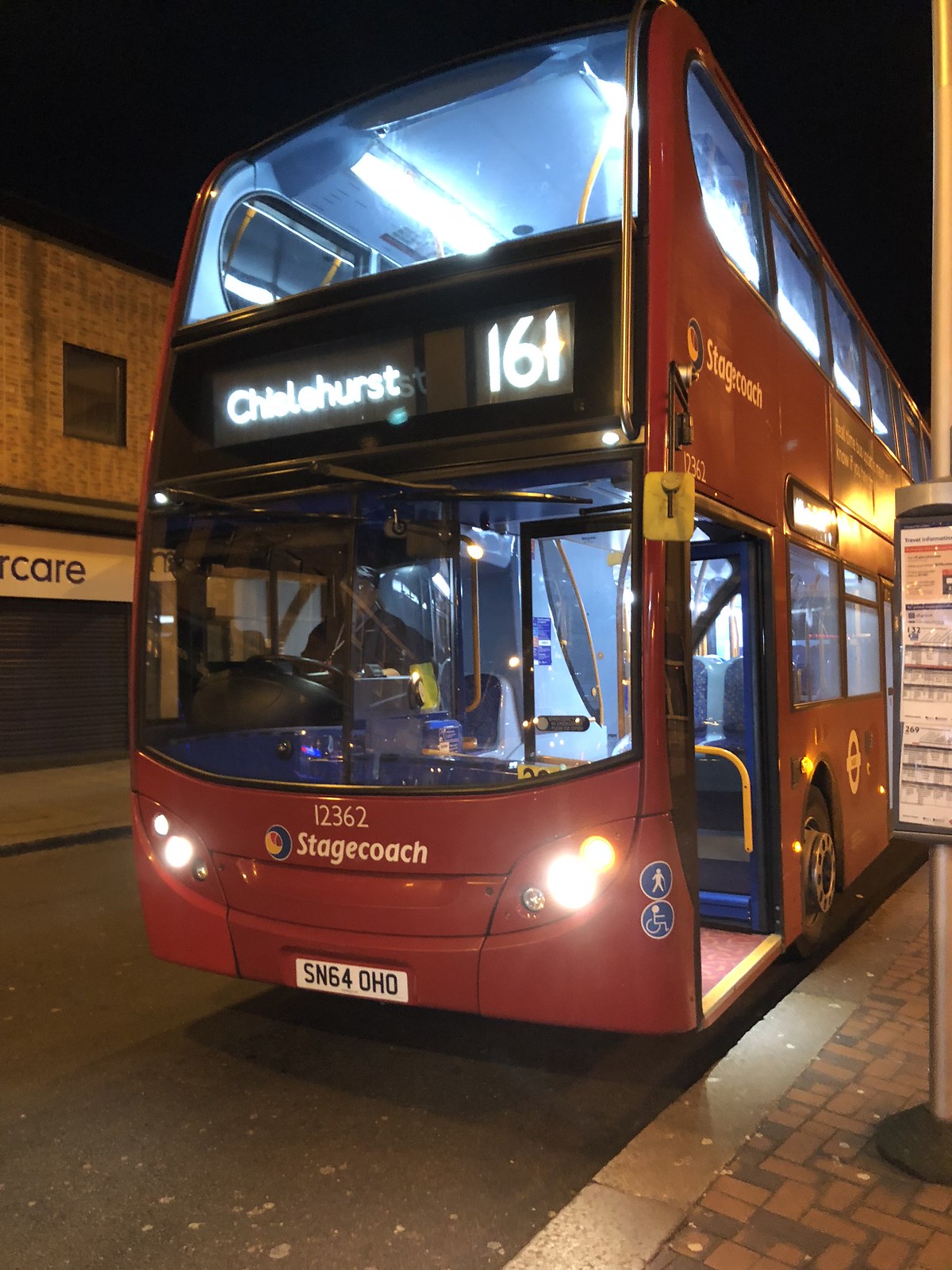This detailed nighttime photograph captures a vibrant red double-decker bus navigating the narrow streets of England. The bus, identifiable by its illuminated sign above the driver that reads "Chislehurst 161", is parked by a sidewalk at a bus stop. The bus's entry door is open, inviting passengers to board, though both decks appear empty. On the bus's front, prominently displayed, is the number 12362 along with the "Stagecoach" business logo. The vehicle's license plate, SN64 OHO, is visible beneath the windshield.

The scene reveals the bus's well-lit interior, illuminating both the lower and upper decks. The image focuses on the bus's front and right portions, highlighting features such as the large windshields, windshield wipers, headlights, and a side logo depicting a standing man and a man in a wheelchair near the entry door.

To the left, a brick building features a white banner with the partially visible word "CARE" and a closed black garage door below it. A brick-paved sidewalk occupies the lower right corner of the photo, while a pole with a partially visible sign stands next to the bus. The backdrop of the scene is a dark, black sky, accentuating the bus's presence in this nocturnal urban setting.